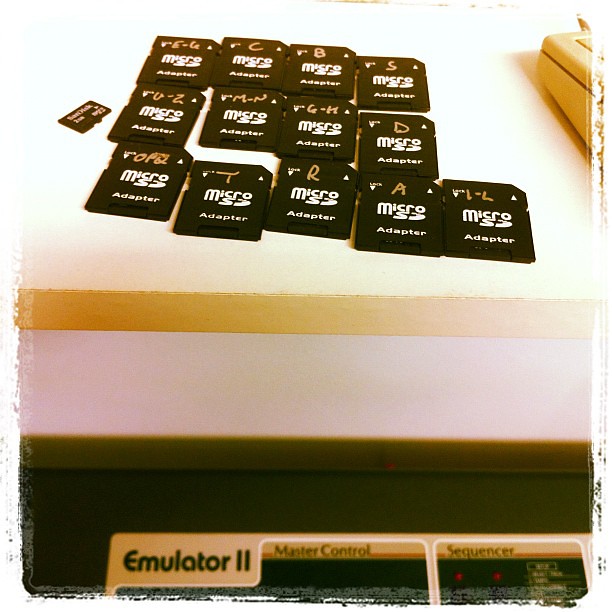The image showcases a cluttered scene on a white desk, featuring thirteen black micro SD card adapters, each labeled with a unique combination of letters including FBBDRGHRAL, E6, C, B, S, V through Z, M through N, G through H, D, O, P, T, R, A, and I through L. These adapters are arranged in three rows, with the top two rows having four adapters each, and the bottom row containing five. Adjacent to the rows of adapters is a smaller SanDisk mini SD card. Below the desk, partially visible, is a machine with the text "Emulator 2, Master Control, Sequencer" written on it. The overexposed photograph renders the wooden texture of the desk almost completely white behind the black adapters.